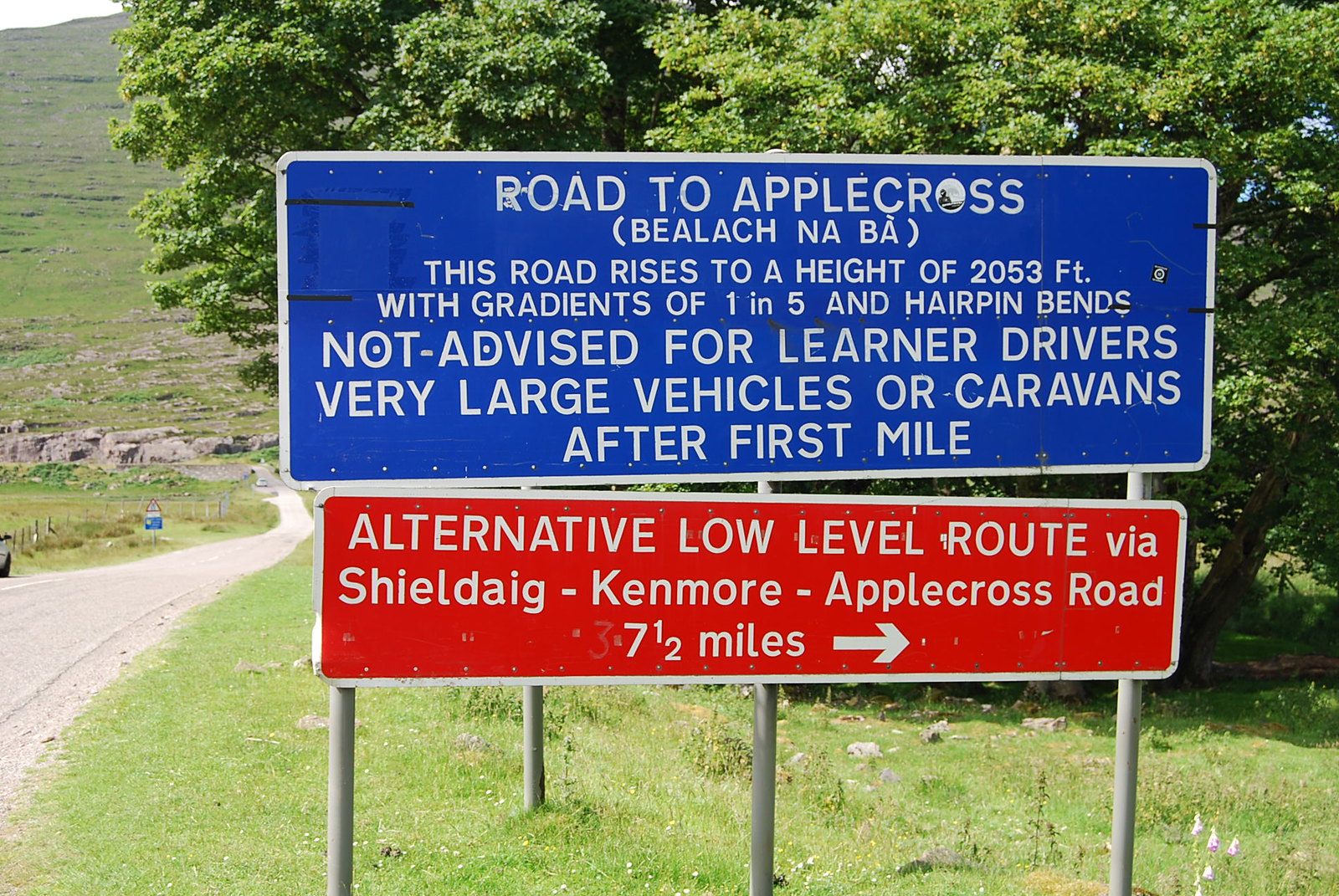The photograph captures an outdoor setting featuring two stacked road signs supported by four metal posts. The top sign is royal blue with white text that states, "Road to Applecross. Bealach na Bà," and provides a cautionary message: "This road rises to a height of 2,053 feet with gradients of 1 in 5 and hairpin bends. Not advised for learner drivers, very large vehicles, or caravans after the first mile." Below it, a red sign with white text offers an alternative route: "Alternative low-level route via Shieldaig-Kenmore-Applecross Road, 7.5 miles," with a rightward-pointing arrow. The background features a grassy area with large trees, and to the left, a roadway stretches into the distance, winding around a hill.